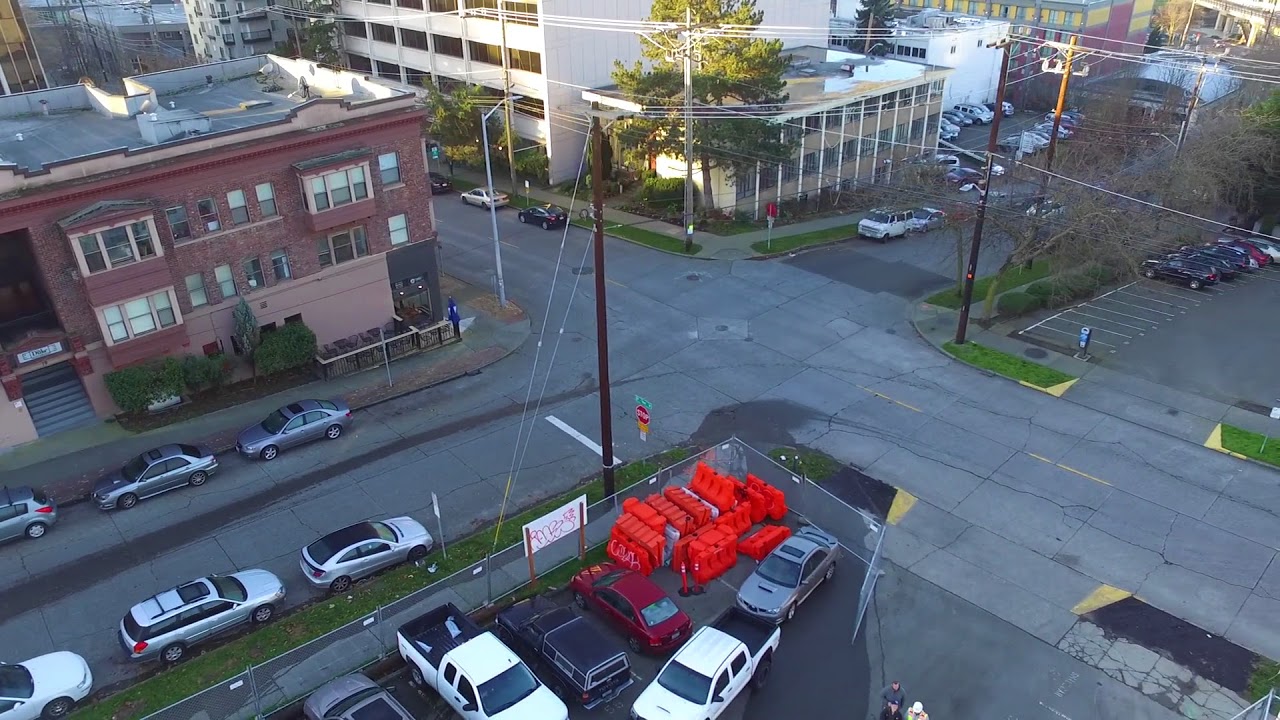This aerial image captures an urban intersection at a standstill, surrounded by a network of buildings and parked cars. The asphalt street, marked by prominent yellow lines and etched with numerous cracks, forms the focal point. Towards the bottom of the frame is a fenced-off area, containing a pile of orange safety barriers and framed by a chain link fence. On the left side within this fenced area, a white sign adorned with graffiti stands supported by wooden boards. Adjacent to this, a power pole festooned with power lines extends in multiple directions.

In the bottom left corner, a three-story brick building with a dark archway entrance and light gray stairs is prominently visible, flanked by a small walkway. Centered in the background is a towering white structure, whose summit is obscured, joined by another white and gray building with a flat roof to its right, followed by a yellow and red brick edifice further back.

On the right side of the image, two parking lots can be seen - one half-filled with cars and the other with some empty spaces. Situated along the sides of the street are numerous parked cars, giving a somewhat residential feel to the area. The scene is brightened by daylight, and two stop signs are visible, facing one direction, with two pedestrians walking at the bottom of the image. Overhead, power lines crisscross the scene, enhancing the urban landscape's intricate detail.